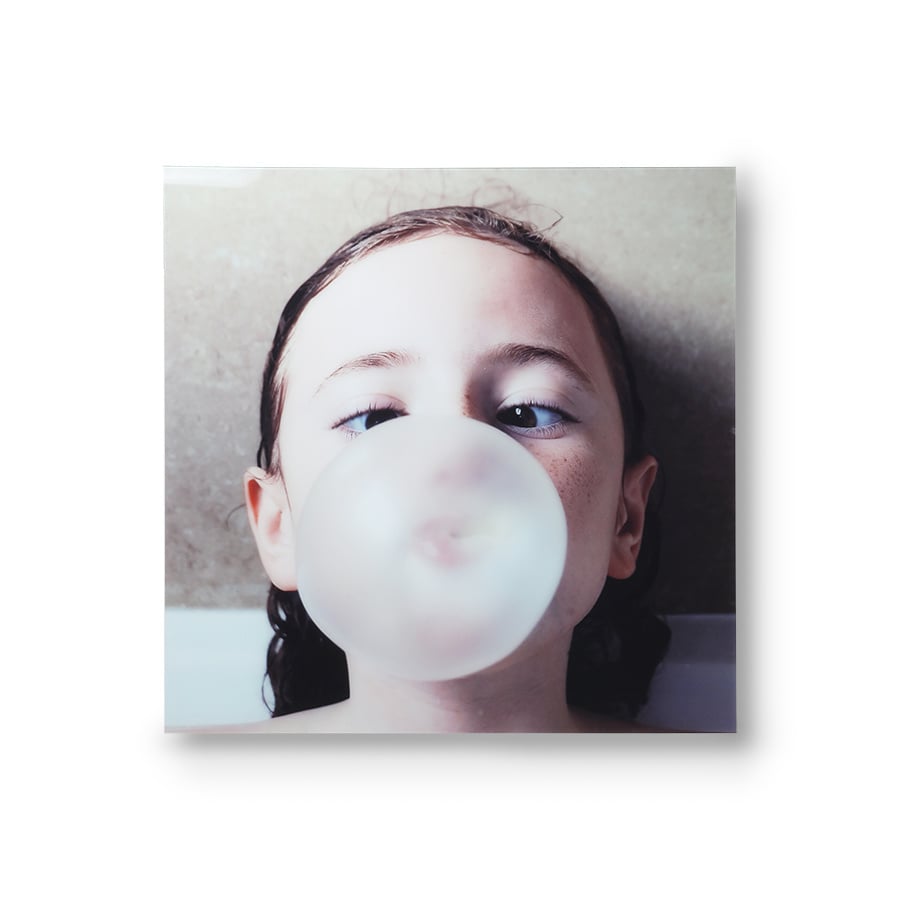This artistic photograph captures a young girl, likely in her early teens, with brown hair pulled back to reveal her ears, and deep brown eyes that are humorously crossed as she focuses on the enormous bubble of pink bubble gum she's blowing. The bubble, nearly white at its peak size, envelops her mouth, chin, and nose, making it the central feature of the shot. Her hair, damp and falling to her shoulders, suggests she may have just come out of the bath. The portrait, framed in a square format, is set against a light brown, grainy background, enhancing the whimsical and professional feel of the image. Her freckled face and playful expression lend a charming touch to the overall composition.